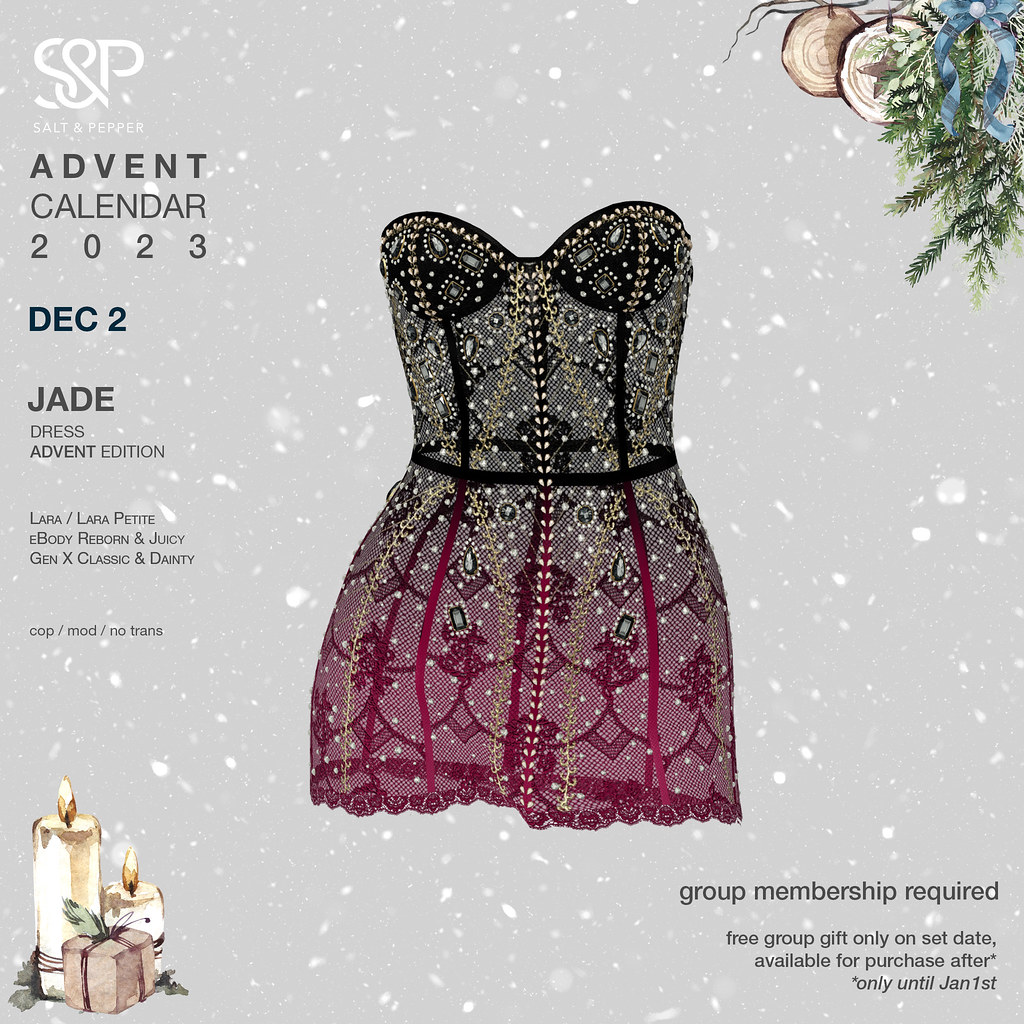The flyer for the Jade Dress Event has a light gray background with a wintry theme, featuring snowflakes throughout. In the upper right corner, there are evergreen branches and wooden ornaments, enhancing the festive atmosphere. At the center of the flyer is an elegant strapless dress with a striking combination of black, yellow, white, and a bold red stripe at the bottom, adorned with intricate black lace details.

The flyer is themed around the Salt & Pepper brand's 2023 Advent Calendar, which is noted at the top left, along with the brand's white logo. The dress in the image showcases a gradient from black at the top to a rosy pink shade at the bottom, interwoven with golden threading and bejeweled embellishments.

Additional details on the flyer include text on the left side, announcing the date of the event as December 2nd, and stating "Jade Dress Advent Edition," along with information about compatibility with various body types like Lara, Lara Petite, E-body Reborn, and more. At the bottom left, there are two candles and a gift box wrapped in brown paper, adding to the seasonal charm. The flyer also mentions that group membership is required and that free group gifts are available only on the event date, with additional purchases available until January 1st.